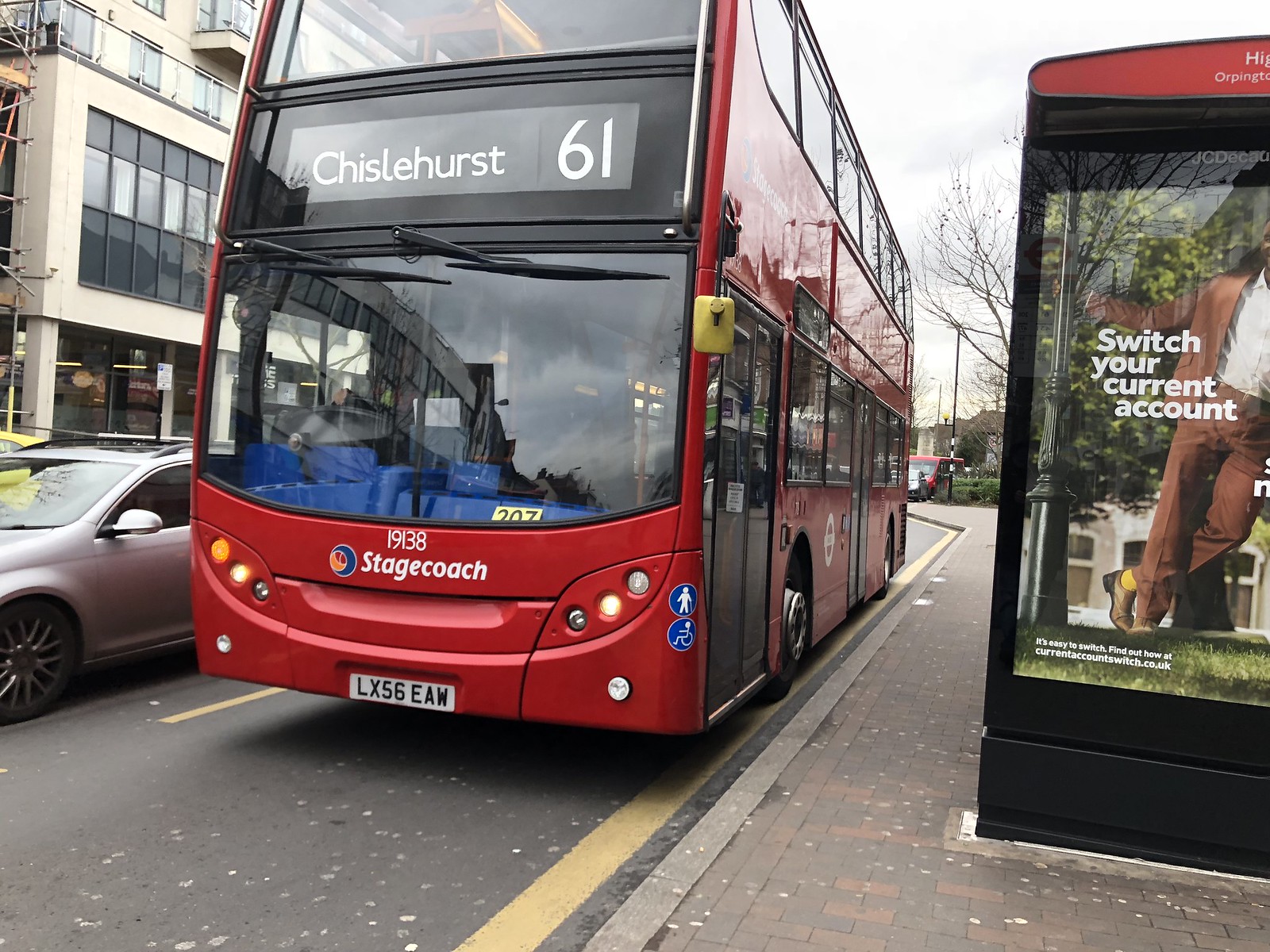The image depicts a bustling London street with a red double-decker bus prominently in the center, facing the camera. The bus, marked "Chesilhurst 61" at the top and "Stagecoach" underneath, has the license plate LX56 EAW. Positioned to the left of the bus is a gray car, while on the right side, a cobblestone sidewalk leads to a bus stop canopy with a red top and black base. Adorning the bus stop is a poster that reads "Switch your current account," featuring an image of a man holding a streetlight. Additional details on the bus include the number 19138 and a symbol indicating handicap assistance. The scene is set in a downtown area with buildings featuring many windows on the left side and cloudy skies overhead, suggesting a typical day in the city.